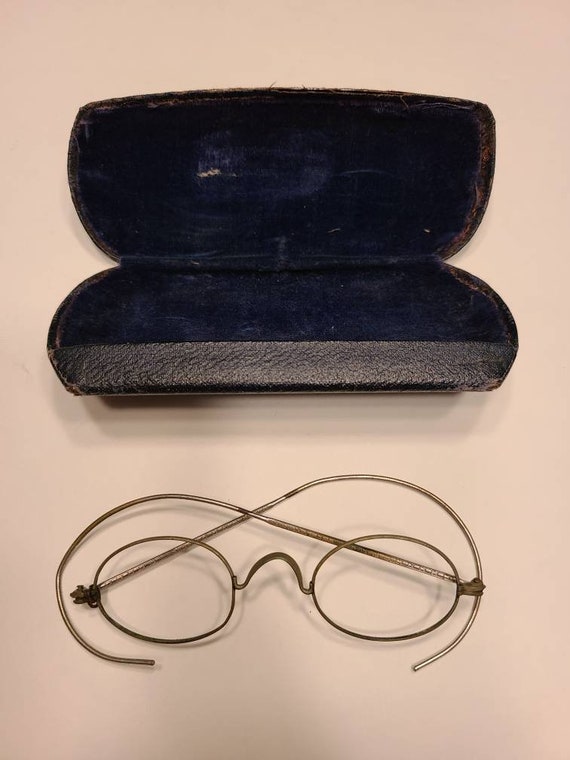This detailed photograph captures an antique eyeglass set displayed on a creamy white-beige surface. The top half of the image showcases an old, worn-out eyeglass case, designed in a dark blue or burgundy, velvety material. The case is noticeably aged, with rusted edges and plucked fabric, adding to its vintage charm. The inner lining comprises a black or dark blue velvet, juxtaposed against a fuzzy white material along the bottom strip, and shows signs of heavy wear with white scratches scattered throughout. The bottom half of the image features a pair of wireframe eyeglasses, estimated to be 40-50 years old. These glasses, missing their lenses, exhibit a bronze or copperish hue, further emphasizing their antiquity. The arms of the glasses, designed to fit over the ears, are asymmetrical and crudely curved, resembling overlapping question marks. Despite their age, the earpiece holders remain intact, crafted from thin, slightly rusted metal, bound to the frame by what appears to be leather or twine. The picture beautifully encapsulates the essence of vintage eyewear, highlighting the passage of time through the intricate details and aged textures.